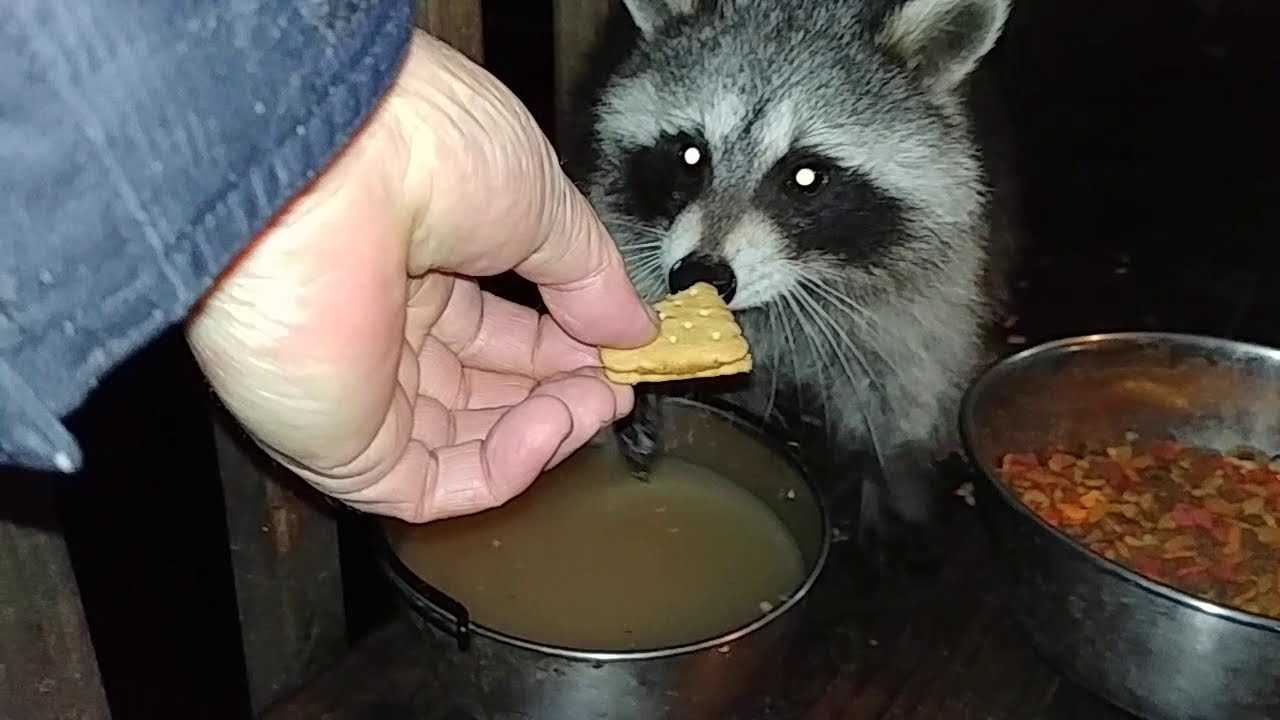In this nighttime photograph, a raccoon with distinctive black markings around its eyes and gray and white fur is the central focus. The raccoon, positioned slightly off-center to the right, is seen sniffing a large tan cracker being held out by a person whose hand emerges from the left. The person's hand, with peach-colored skin and a slate-blue cuff, extends towards the raccoon's snout. Below the raccoon, there are two steel-colored pots: one to the bottom right containing what looks like animal kibble, and another to the left-center filled with a discolored liquid, possibly muddy water or some kind of broth. The scene, enveloped in darkness, leaves the surroundings largely in shadow, making the feeding interaction the primary highlight.